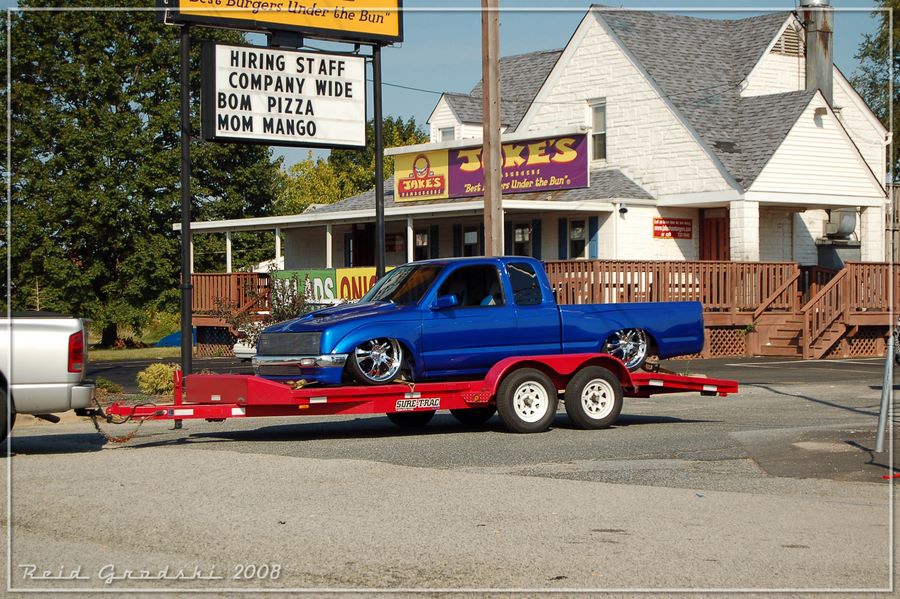In this daytime photograph with clear, beautiful blue skies, a customized deep blue pickup truck is being towed on the back of a red trailer, which is hooked to a gray pickup truck parked on the street. This scene unfolds in front of an establishment, possibly a restaurant or business, called Jake's. The establishment is housed in a white building styled like a house, surrounded by an extensive brown wooden fence and marked with a predominant sign that reads "Jake's" in yellow letters on a blue and red backdrop. Another sign, slightly visible and white with black lettering, announces "Hiring Staff Company-Wide - BOM Pizza, MOM Mango." Notably, in the upper left corner, a large tree with lush green leaves adds a touch of nature to the scene. Additionally, the lower left corner of the image features the text "Reed Grodzki, 2008," indicating the photographer or date.